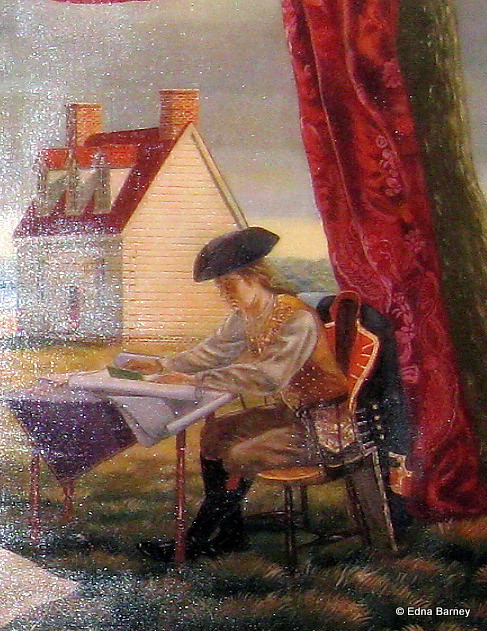This image captures a meticulously detailed painting, likely an oil painting, depicting a colonial-era man seated at a desk outdoors. The man wears a distinctive black tricorn hat and has long hair pulled back into a loose ponytail. His attire includes a gold-colored vest over a white shirt with puffy sleeves, tan pants, and knee-high black boots. Draped over the back of his wooden chair is a notable black coat with red lapels and gold trim, featuring five buttons in a vertical row, indicative of a military long waistcoat jacket from the colonial period.

The man is intently examining papers spread out on the table, which appear to be plans or blueprints, hinting at his engagement in some form of design or construction. The table, covered with a cloth, and the wooden chair are placed on a grassy patch, enhancing the outdoor setting. To his left stands a tree with striking red foliage in the foreground, with its darker branches receding into the background. 

In the backdrop, there is a white boarded building with a red A-frame roof, featuring three windows each topped with their own A-frame peak and flanked by two red brick chimneys at either end. A tall red curtain extends from nearly the top to the bottom of the image behind the chair, and gray, ominous clouds loom in the sky above the house, adding a dramatic atmosphere to the scene. The bottom right corner of the painting includes the signature "Edna Barney" in white lettering, indicating the artist's credit.